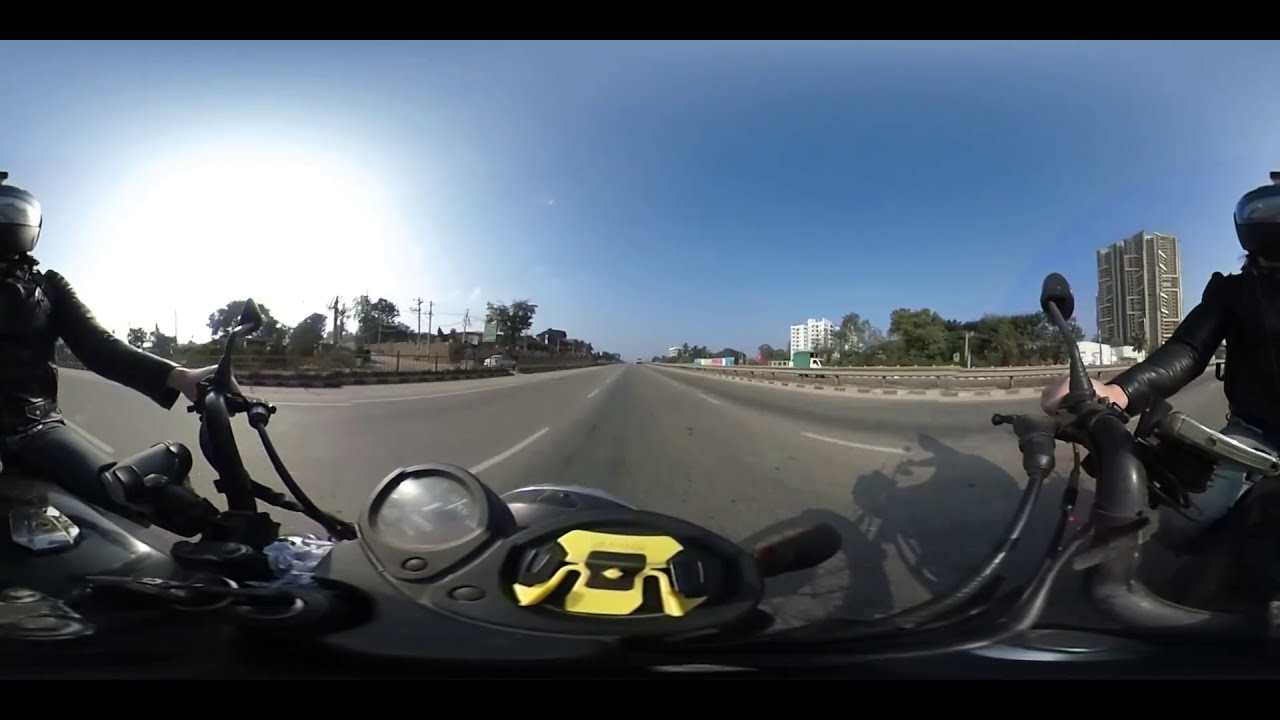This detailed panoramic photograph, taken from the perspective of a motorcyclist, showcases a vibrant three-lane highway under a rich blue sky. The foreground prominently features the black handlebars and console of the motorcycle, situated at the image's center. To the immediate left and right, the photograph appears to create a surreal, duplicated effect, revealing two other motorcyclists in black attire; one on the left, sporting a matte black helmet and blue jeans, and another on the right, both of whom ride black motorcycles. The highway itself is dark gray with clear white lane markings. Alongside the road, low metal barricades and safeguards are visible, giving way to an elevated view of trees and telephone poles on the left, and greeneries and apartment high-rises on the right. The backdrop of the scene is lit by a glowing white sun in the left side of the unmarred, bright blue sky. The setting sun adds a distinctive sheen to the image, emphasizing both the clear day and giving the entire photograph a slightly dreamy, distorted essence typically seen in wide panoramic shots.